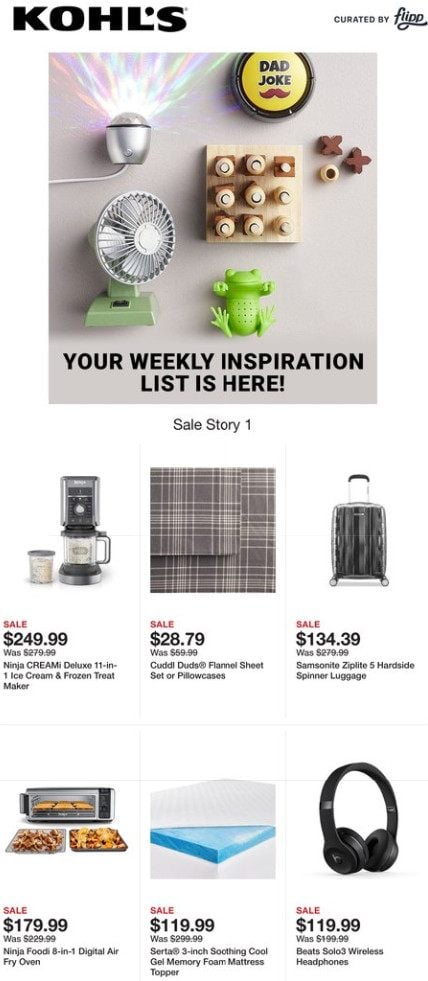This is a detailed and descriptive caption for the image:

---

This image is a cropped screenshot of a Kohl's advertisement designed to showcase curated products by Flip. At the top of the ad, the Kohl's logo is prominently displayed in large black letters, with the phrase "curated by Flip" in smaller black letters to its right. The central focus of the advertisement is a large, square thumbnail image, taken from an overhead perspective, featuring an array of various products neatly arranged on a table.

Below this main image, the ad features the phrase “Your Weekly Inspiration List is Here” in bold black letters, signaling new product selections. Beneath this, the words “Sales Story One” are written in small black letters, likely indicating a thematic sales event.

The lower section of the image is dedicated to six product thumbnails, arranged in two rows of three. Each product listing begins with a thumbnail image at the top, followed by the word "Sale" in bold red letters. Directly underneath the "Sale" label, the current sale price is shown in bold, followed by the original "was" price, which is also displayed for comparison. Each product has a brief description written below the pricing information.

The first product featured is the Ninja Creamy, offered at a sale price of $249.99, down from its original price of $279.99. The product description reads "Ninja Creamy Deluxe 11-in-1 Ice Cream and Frozen Treat Maker" in small black letters. The remaining five products span various categories, each with its own dedicated thumbnail, pricing details, and brief descriptions.

---
This detailed caption aims to thoroughly describe the content and layout of the Kohl's advertisement for clear understanding.